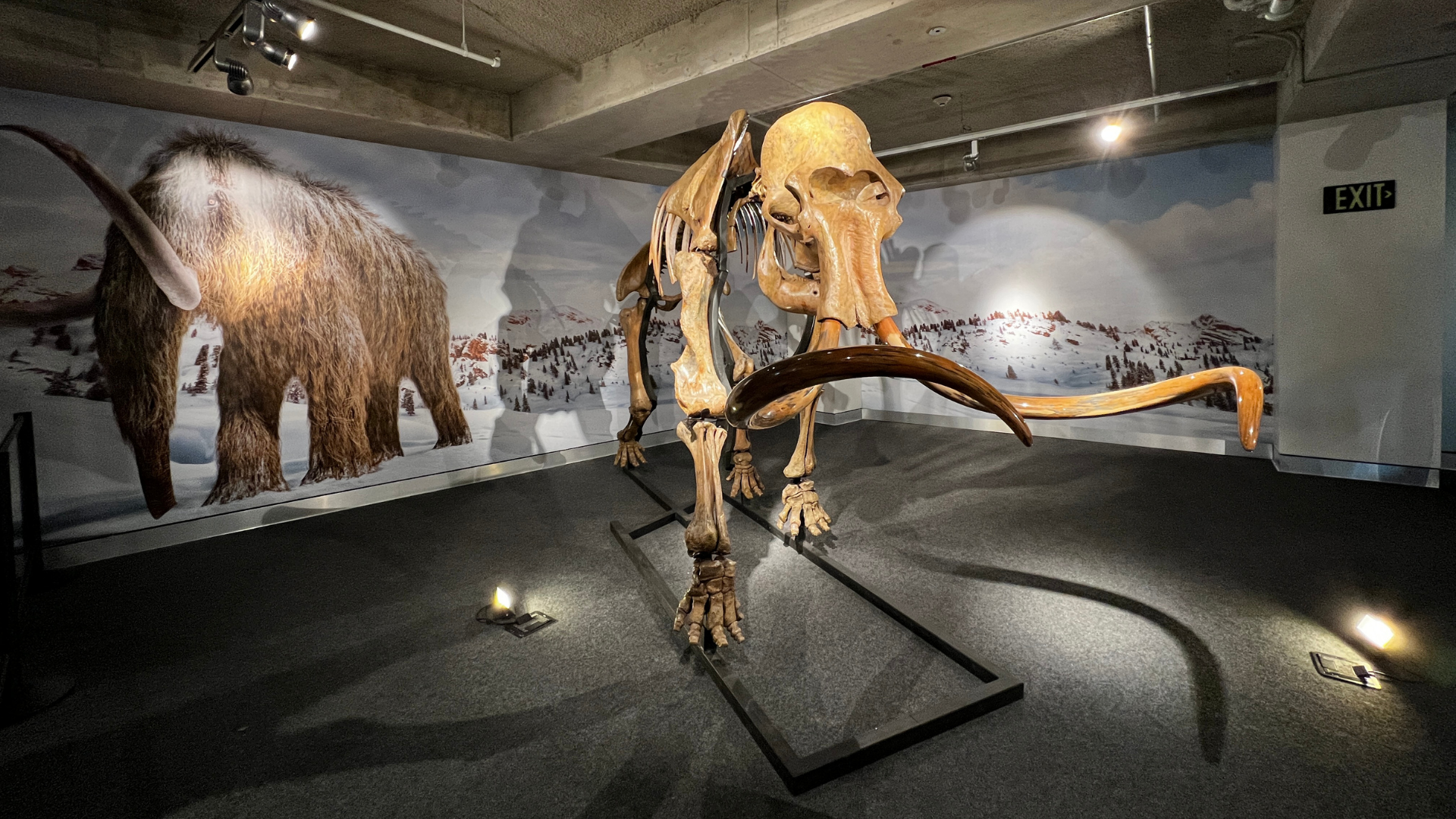In this photograph showcasing a museum exhibit, we observe the skeleton of a colossal mammoth standing prominently within a spacious room, illuminated by multiple spotlights. The skeletal remains exhibit an ivory hue, with enormous tusks extending to the right. The display rests on a black, speckled carpeted floor, accentuated by upward-facing lights.

Encircling the room’s perimeter is an expansive mural that vividly recreates the mammoth's natural habitat. This mural features a winter landscape, complete with snow-laden trees and rolling, snow-covered hills that wrap around the room, creating an immersive diorama. The left-hand side of the mural contains an artistic depiction of a woolly mammoth in its full, fur-covered majesty, walking through the snowy environment. The room is adorned with a concrete ceiling, from which additional lights hang, further highlighting the mammoth skeleton. In the corner, an 'exit' sign can be spotted among the other illuminations, subtly integrating functionality with the exhibit's grandeur.